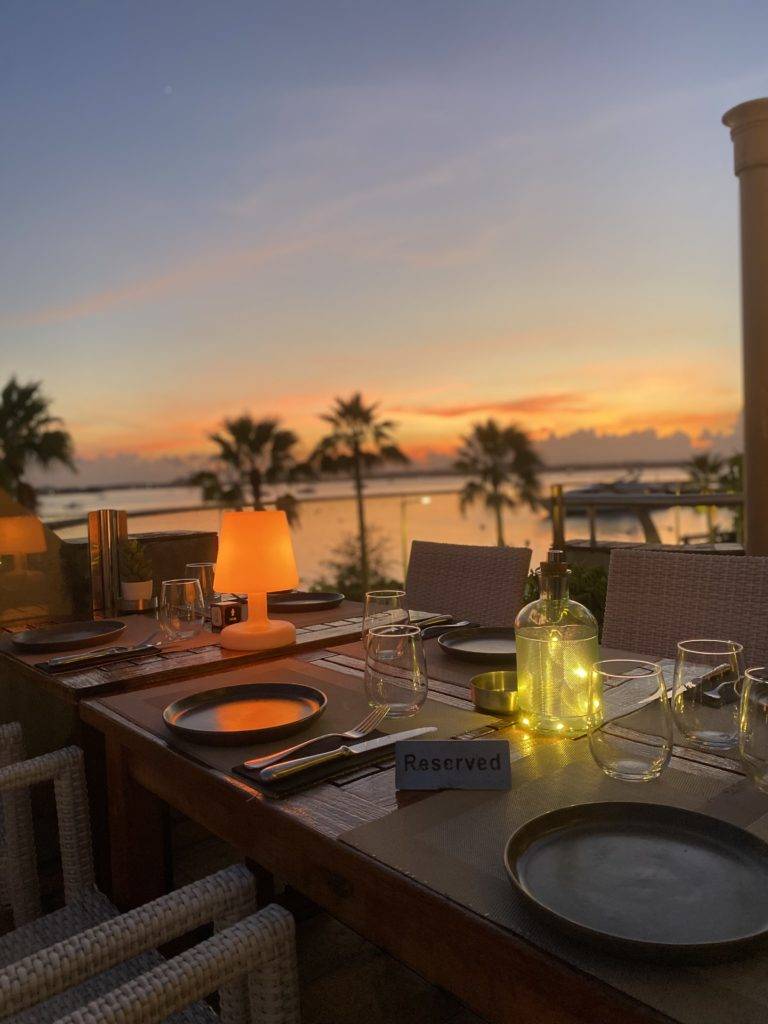The image captures an elegantly set dinner table situated on an outdoor patio of a restaurant, clearly marked with a white "Reserved" sign in bold black letters. The table, appearing to be two square tables pushed together, is adorned with placemats, plates, silverware, glass drinking glasses, and a lantern lit with a candle, adding a cozy illumination alongside a small, glowing white lamp. Surrounding the table are gray, wicker-like chairs, positioned for an inviting dining experience. In the foreground, the well-arranged dining setup sharply contrasts with the breathtaking natural backdrop. The distant view showcases palm trees swaying gently in the breeze against the backdrop of an expansive ocean. The sky above transitions from a serene blue to a warm, glowing gradient of oranges and yellows, suggesting a picturesque sunset over the water, enhancing the idyllic atmosphere reminiscent of a beachside restaurant, possibly in a setting like Los Angeles.